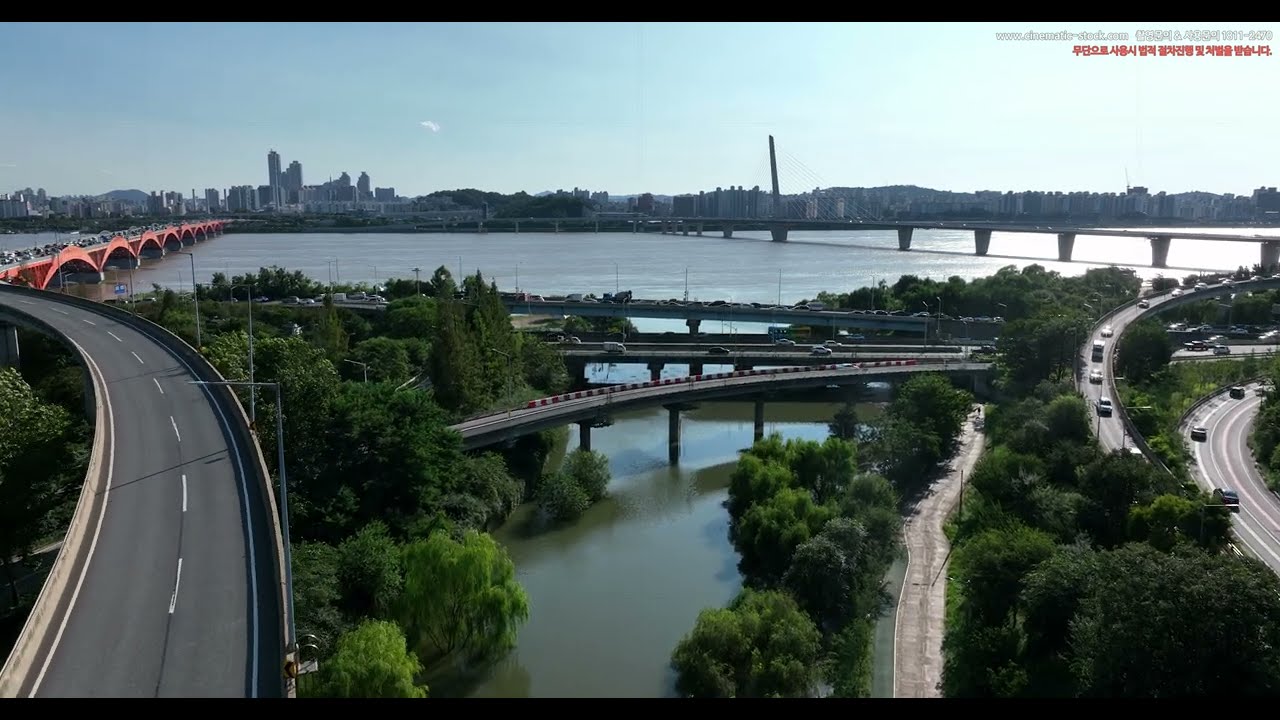This aerial photograph captures a complex urban landscape defined by a network of bridges and roadways interwoven with bodies of water and greenery. Several bridges, their pillars towering around 30 to 50 feet high, crisscross over a lake, creating a sprawling web of highways and arterial roads. One prominent bridge, distinguished by its red arches, is heavily trafficked and arcs across the lake, seamlessly connecting to the city's outskirts. Adjacent to this red-arched bridge is a gray bridge, illustrating the varied infrastructure leading into the expansive city of skyscrapers on the horizon.

Closer to the camera, a series of smaller bridges span a twisting smaller river, with lush clusters of trees interspersed throughout the landscape. There is also a looping road visible among the greenery. Near the lower right side of the image, a dirt path inclines towards a freeway, indicative of pedestrian walkways amidst the natural setting. The photographic setting is during a bright, sunny day as indicated by the light blue sky overhead. Collectively, the image depicts a harmonious blend of nature and urban development, marked by intricate transport connections converging towards the distant, bustling metropolis.